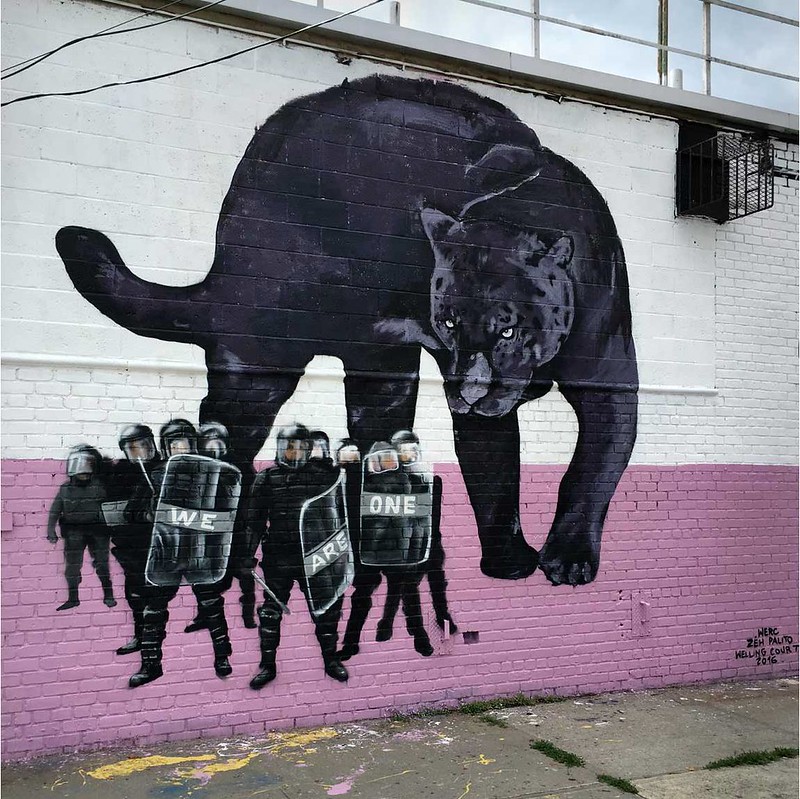This photograph captures an incredible graffiti mural on the side of a brick building. The building's base third is painted dusky deep pink, transitioning to white for the top two-thirds. Set against this vibrant backdrop, a large black panther prowls ominously, taking up a significant portion of the wall. Below this, in the bottom left, stands a squad of nine SWAT officers in black riot gear, complete with helmets and shields. Their shields bear the collective message, "We Are One" in white letters. Above the mural, a white metal fence and some hanging wires are visible, along with a small black cage-like structure on the right. The ground in front features large cement blocks interspersed with grass and weeds. At the bottom right corner of the pink wall, partial black writing appears, though only "Welling Court" is discernible.